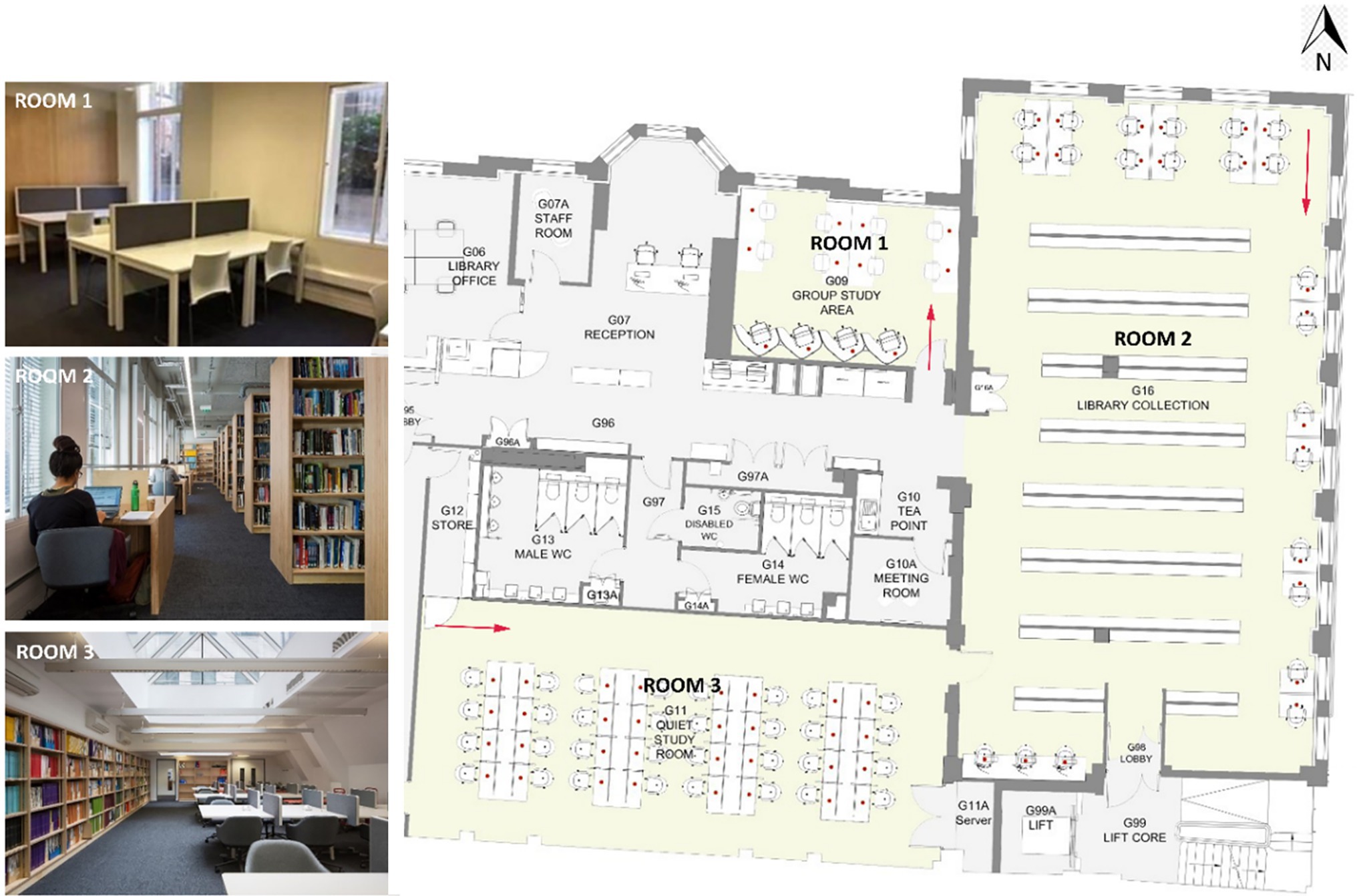The composite image displays a detailed layout of a library, consisting of three smaller photographs aligned vertically on the left and one larger schematic on the right. The first image, labeled "Room 1," portrays a study area with two large beige tables, each divided by black separators, and beige chairs. The room features dark carpeting, a pair of large windows revealing a bright outdoor view with trees, and baseboard radiators. The second image, labeled "Room 2," shows a well-lit library space lined with bookshelves on the right and desks with students working on laptops on the left. It has large windows and a long fluorescent light overhead, with dark gray carpeting. The third image, labeled "Room 3," captures a section of the library with long bookcases recessed into the wall, gray study desks with separators, and a ceiling with beams allowing natural light to flood in from a large skylight. The larger image to the right is a floor plan of the library, detailing the locations of Rooms 1, 2, and 3, as well as various other areas such as a reception, staff room, library office, meeting room, and restrooms. Room 1 is indicated to be a group study area, Room 2 a library collection room with study carousels and a lift core, and Room 3 a quiet study space. Each section of the library and its function is clearly marked, providing a comprehensive overview of the building's layout.